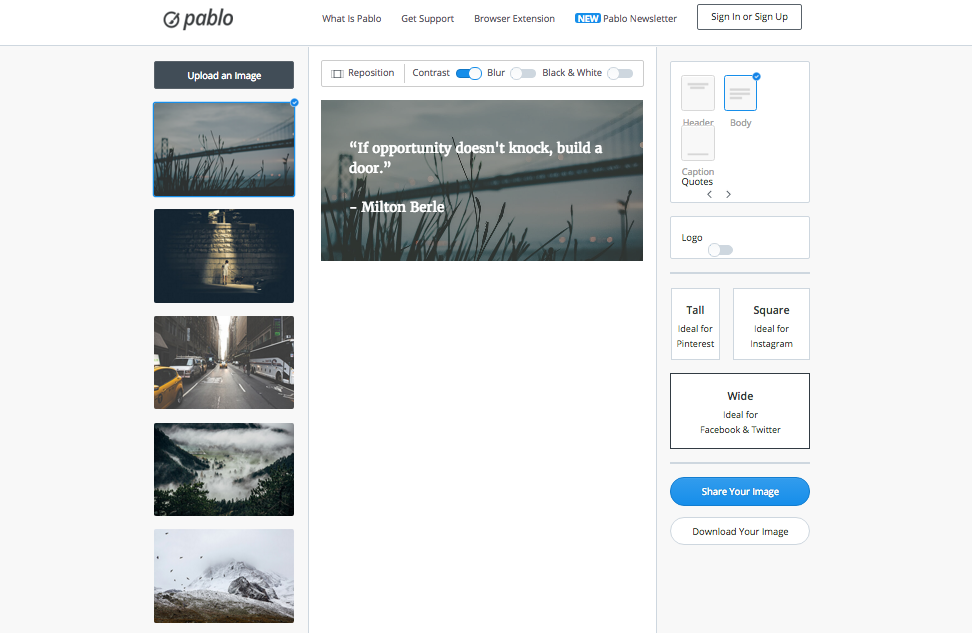The image depicts a screenshot of a photo editing software called Pablo. On the left side of the interface, the word "Pablo" is written in black text, accompanied by a check mark. Below it, there's an option labeled "Upload an Image." Beneath this, five image thumbnails are displayed in a vertical arrangement:

1. The first image features a bridge, partially obscured by reeds or tall grass.
2. The second image shows a wall illuminated by sunlight streaming in.
3. The third image captures a bustling street scene that appears to be in New York City.
4. The fourth image depicts waves crashing against rocky shores.
5. The fifth image reveals a snowy landscape atop a mountain.

To the right of these thumbnails is a prominent picture with the text "If opportunity doesn't knock, build a door" written in white, centered on the image. Above this picture are several editing buttons labeled "Reposition," "Contrast," "Blur," and "Black and White."

On the far right side of the interface, there is a column of symbols and labels denoting different layout options: "Header," "Body," "Quotes," "Logo," "Tall," "Square," and "Wide." Below these options, there is a call-to-action button with the options "Share Your Image" or "Download Your Image." The overall layout and features indicate a user-friendly tool designed for creating and customizing visual content.